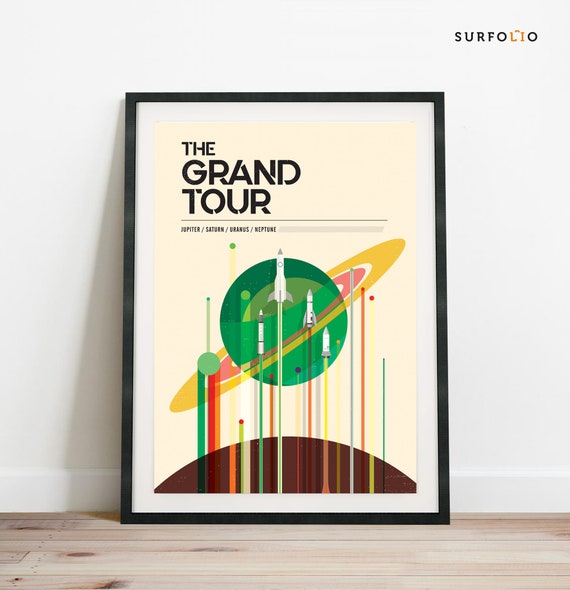A framed artwork titled "The Grand Tour: Jupiter/Saturn/Uranus/Neptune" rests on a beige wooden floor against a white wall. In the top right corner, the name "Serfolio" is visible, possibly indicating the brand. The thin black frame encloses a striking computer-generated image showcasing the planet Saturn. Saturn, depicted with a green center and pink and yellow rings, is surrounded by vibrant, colorful streaks in green, red, orange, yellow, and blue. Four distinct rockets are seen flying with trails of different colors: green, light green, red, and yellow. Additional colorful streaks without rockets dynamically radiate across the image. In the lower part of the picture, a brown planet is also visible, adding to the celestial composition.